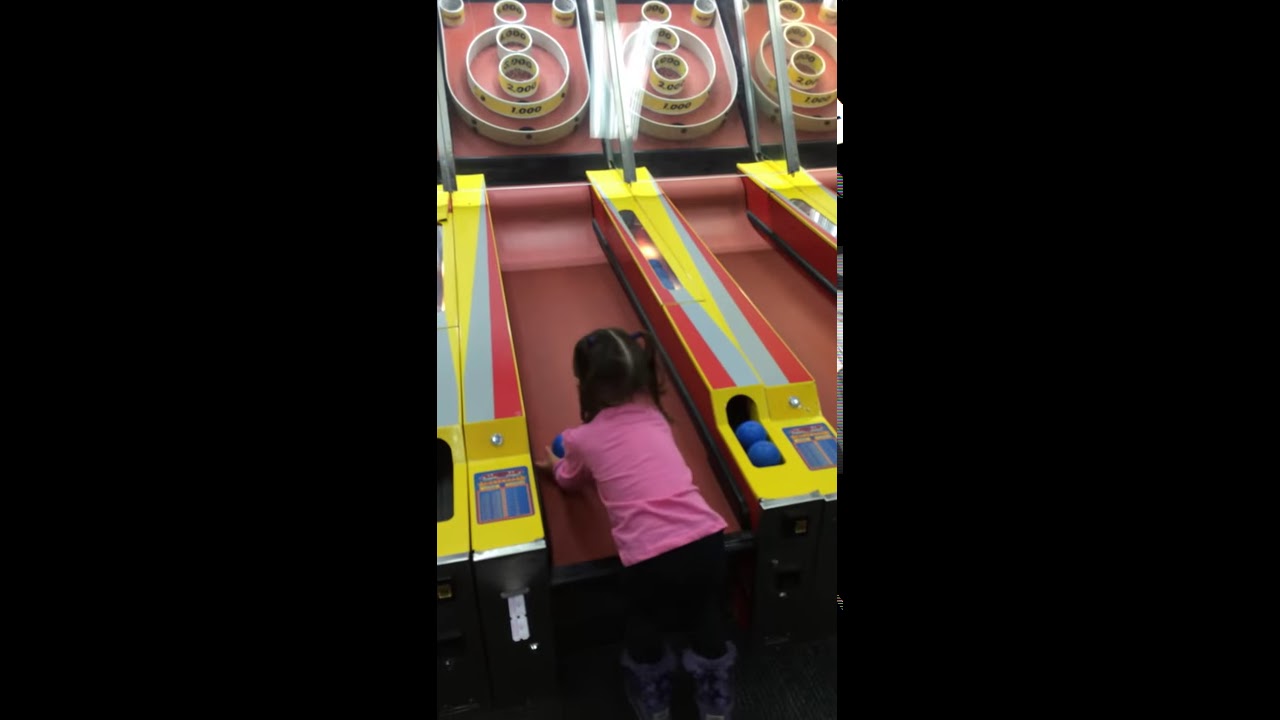In this vivid color photograph set against a solid black background, a young girl, around four years old, is captured in portrait orientation, standing at the forefront of a vibrant ski ball arcade machine. She is positioned centrally at the bottom of the image, leaning over the machine's rampway with a blue ball poised in her hand. Her attire consists of stylish gray fur boots, black pants, and a long-sleeve pink shirt that matches the lively hues of the scene. Her black hair is neatly tied into two ponytails on either side of her head. The ski ball machine itself is colorful, featuring a pink ramp that leads up to circular targets with point values ranging from 1,000 to 5,000. The sides of the machine are adorned with yellow along with light blue and red stripes. Two additional machines are partially visible on the right, contributing to the immersive arcade setting that brings an element of photographic realism to the image.